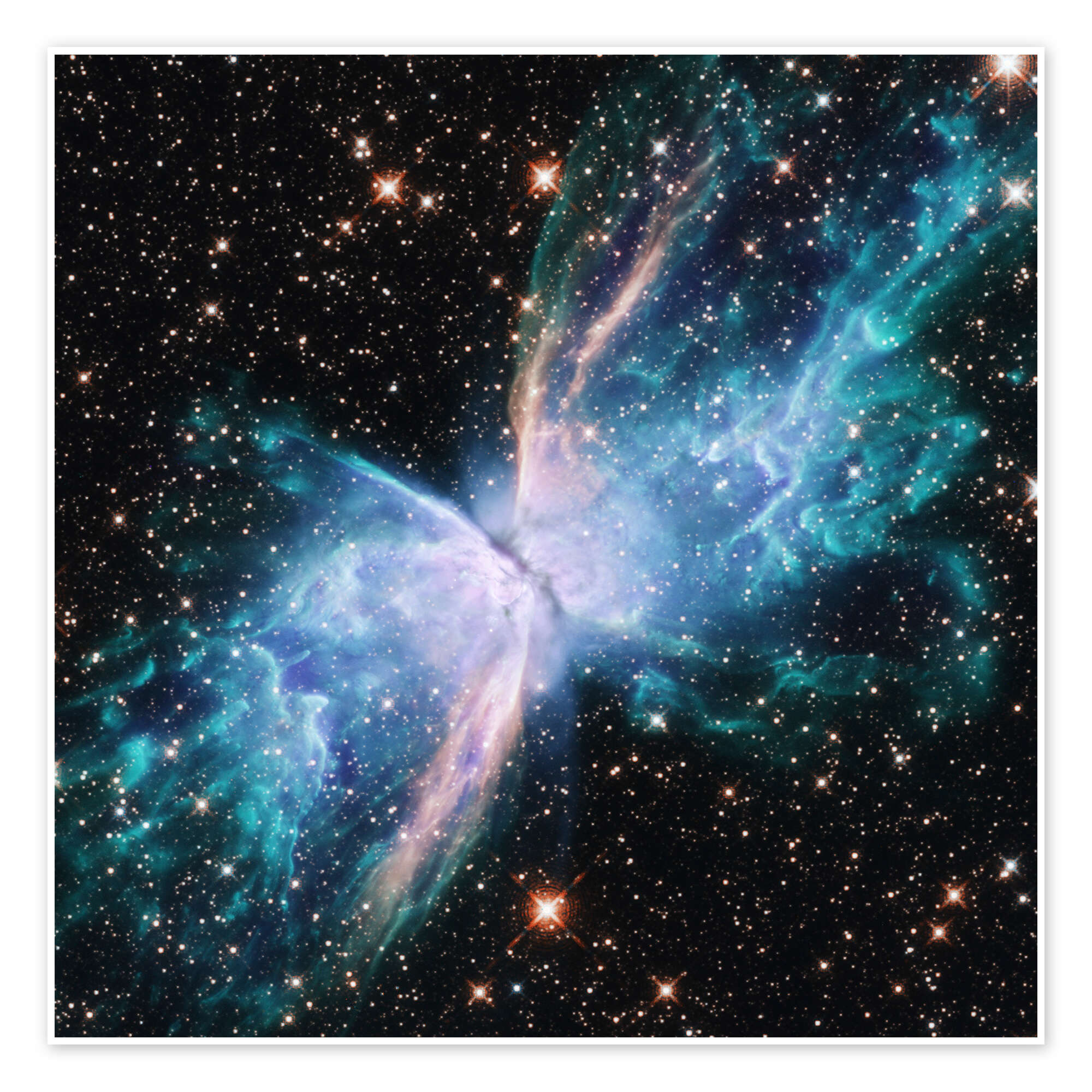This highly magnified time-lapse photograph of a section of the night sky, captured using an advanced telescope, reveals an ethereal butterfly-shaped nebula that dominates the image. The nebula's delicate wings, rendered in striking hues of blue with hints of pink and green, spread out majestically on either side of a darker central structure resembling the body of a butterfly. The center appears lighter and almost gives the impression of antennae extending from it. The surrounding dark sky is studded with countless stars, some of which are captured with rays of light emanating from them, especially the larger ones. The overall scene, with its magical, swirly, and cloudy appearance, evokes a sense of wonder and curiosity about this celestial spectacle.